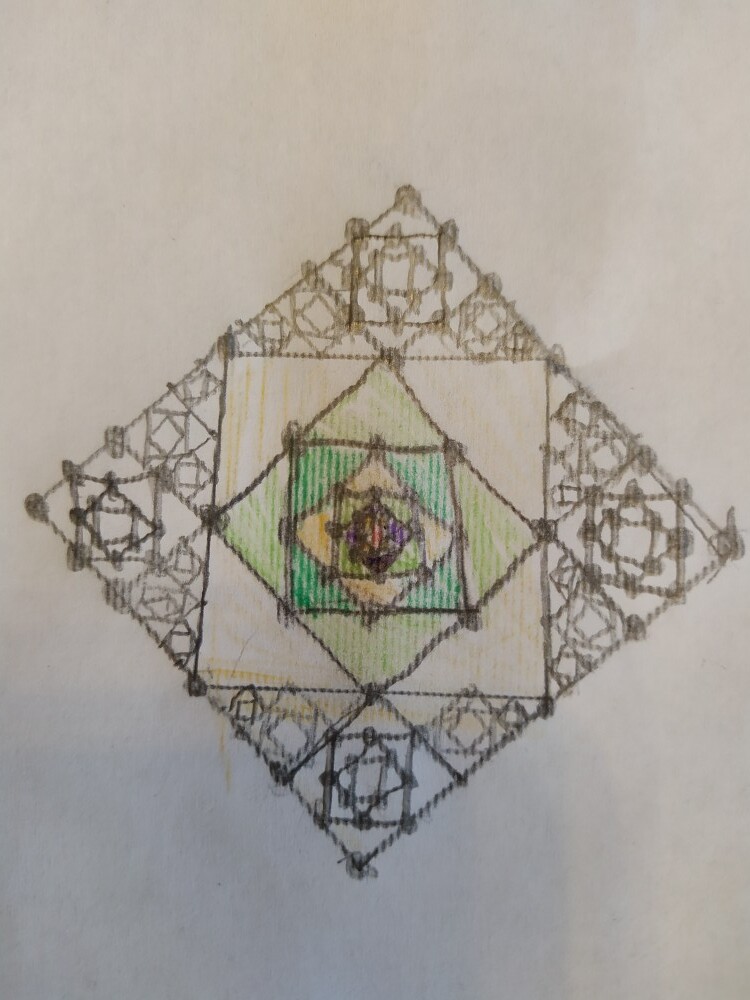This intricate arts and crafts piece showcases a mesmerizing pattern of concentric squares. The composition begins with a large, square gray frame. Within this frame, a series of progressively smaller squares are meticulously arranged. Each subsequent square alternates between a standard square orientation and a diamond orientation (a square rotated 45 degrees). The pattern starts with a diamond-shaped square nested within the large gray frame, followed by another square perfectly aligned within the diamond. This alternating square and diamond schema continues, creating a captivating visual effect that emphasizes precision and repetition. The craftsmanship highlights both geometric harmony and the engaging aesthetic of recursive design.